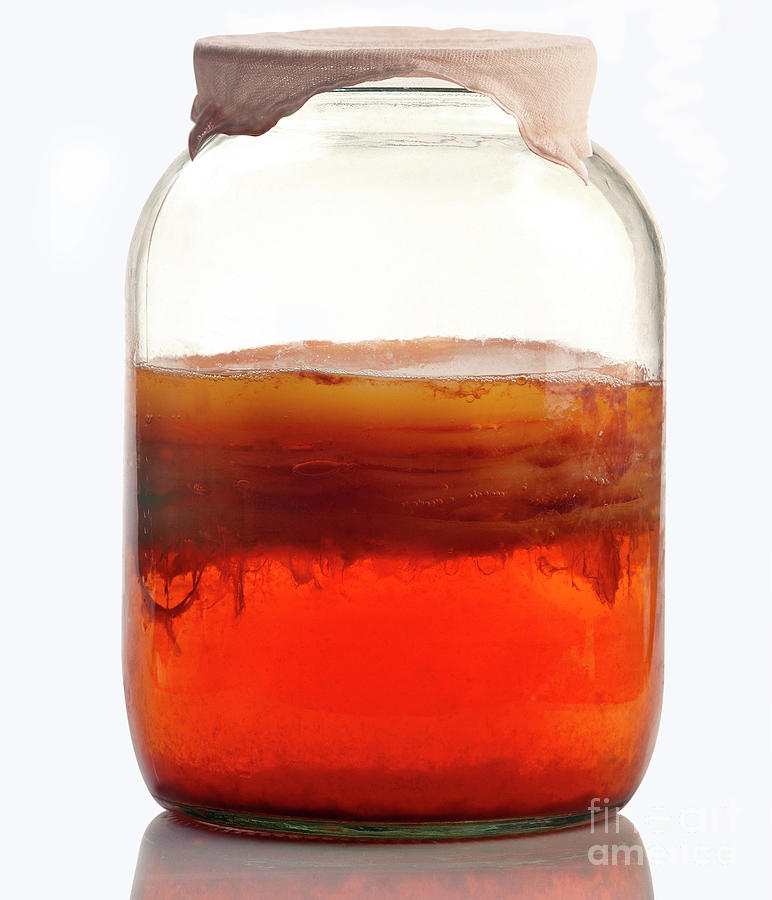This is an image of a clear glass jar in portrait mode, partially filled with a thick liquid that exhibits a gradient of colors. The liquid transitions from a deep red at the bottom, through amber and orange hues, to yellow and brown at the top. The jar has a narrower opening than its full body, which is covered with a white cheesecloth, secured without a lid. The cheesecloth drapes over the top, and there is a solid, gel-like layer on the surface of the liquid, suggesting a fermenting process. The contents of the jar include noticeable streaks and areas of separation, likely indicating layers within the fermenting liquid. Bubbles are visible towards the top, reinforcing the idea that this might be a probiotic drink, such as kombucha. The jar's reflection is subtly visible in the background, and the bottom right-hand corner features the text "F-I-N" over the letters "A-M."